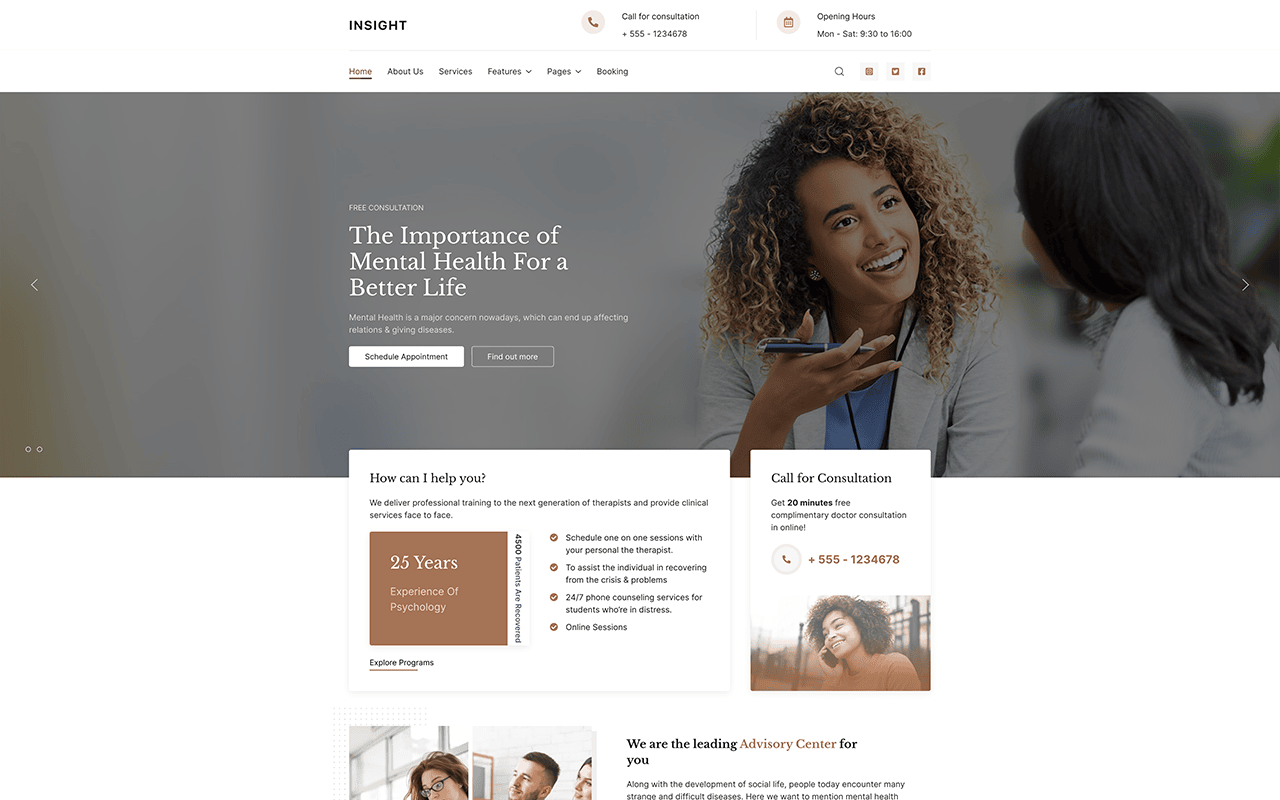The image appears to be a screenshot from a health-related website. At the top left corner, there is the name of the company in bold black font: "Insight." Adjacent to the company name, there is an icon of a phone accompanied by the text, "Call for Consultation," along with a placeholder phone number: 555-123-45678. Further right, there is a calendar icon indicating the operating hours: Monday to Saturday, 9:30 to 16:00.

The top section of the webpage is predominantly white, establishing a clean and neutral starting point. Below this area is a row of navigational buttons. The "Home" button is highlighted in brown, suggesting it is the currently active section. The adjacent buttons, in black, include: "About Us," "Services," "Features," "Pages," and "Bookend." On the right side of this row, there are several icons, presumably for a search function (indicated by a magnifying glass) and social media links such as Facebook and Twitter.

Below the navigation bar is a feature photo displaying two women. One of the women is wearing a doctor's outfit—a white jacket over a blue shirt—suggesting she is a medical professional. She is smiling and engaging with another woman whose head is turned. Overlaying the photo is a text: "The Importance of Mental Health for a Better Life," along with buttons for scheduling appointments and finding out more information.

Further down the page, additional text expands on the services provided: "How can I help you? We deliver professional training to the next generation of therapists and provide clinical services face-to-face." The text is arranged in one or two larger text boxes, with a third box partially visible, indicating more detailed information is available as the user scrolls down.

Overall, the layout is structured to offer immediate access to essential information and navigation, along with a focused message on mental health and professional services.